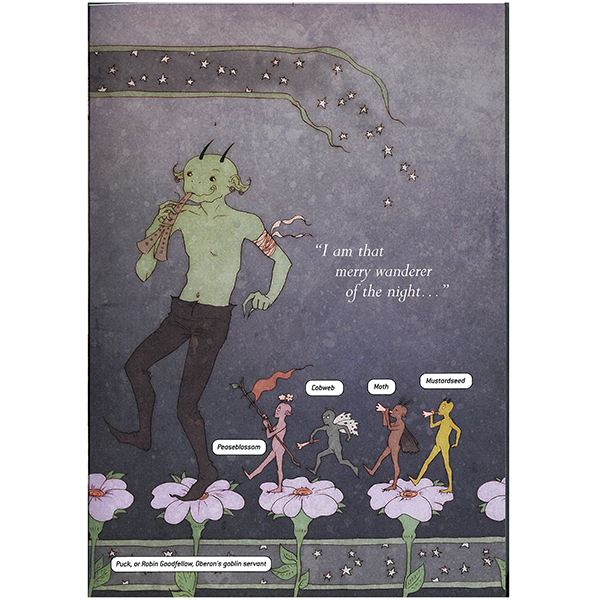This detailed and vividly illustrated image appears to be a scene from a children's book, featuring a whimsical and surreal composition. At the forefront is a green goblin, shirtless with two prominent horns on his head. His left bicep is wrapped in a bloodied bandage, hinting at a recent injury. The goblin holds an unusual object in his mouth, resembling a split wishbone, possibly a type of flute. He marches barefoot across a path strewn with purple flowers, each with green stems and red centers. Above him, a text reads, "I am that merry wanderer of the night."

Following closely behind the central goblin are four distinct, smaller goblins: one pink, one gray, one red, and one yellow. These miniature characters also step on the same flower pathway, their presence adding depth to the whimsical scene. The backdrop is a dark, swirly expanse sprinkled with stars, giving the illustration a magical, night-time atmosphere. Two lines at the top of the image seem to emit additional stars, enhancing the fantastical setting. The overall avant-garde style and rich details make this artwork captivating and enchanting.